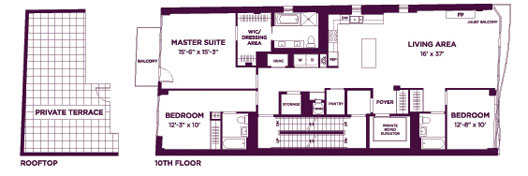The image depicts an architectural plan for a three-bedroom apartment located on the 10th floor. This detailed blueprint includes a main living area combined with a kitchen, offering a spacious and open layout. The living area is fair-sized, providing ample room for various activities and furnishings.

The master suite is generously proportioned and features a large dressing area. It is designed for comfort and convenience, making it an ideal retreat. The second bedroom also includes a private bathroom, offering additional privacy and functionality, which is a desirable feature for residents or guests.

A distinguished foyer serves as the entry point of the apartment, leading seamlessly into the interconnected living area and kitchen. Despite initial confusion, the kitchen is indeed integrated with the living space, forming a cohesive environment for cooking and socializing.

Additionally, the plan includes an annotated rooftop area, depicted separately on the side. This rooftop section is minimalistic, outlined in deep black or brown lines, forming an incomplete rectangle. The center of this rooftop plan features a grid pattern, akin to graph paper, and is labeled "private terrace." This indicates an exclusive outdoor space available for use by the apartment occupants, enhancing the overall living experience with an opportunity for private outdoor leisure.

In summary, this architectural plan showcases a well-thought-out apartment layout with a blend of private and communal spaces, enhanced by the luxury of an exclusive rooftop terrace.